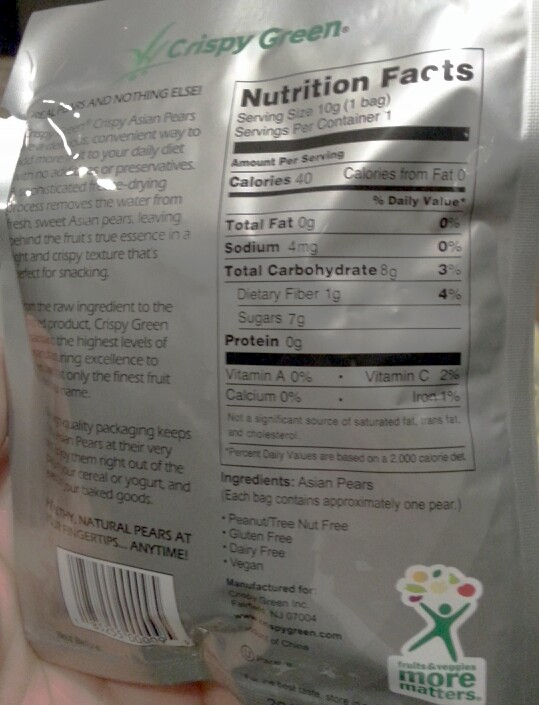Here is a cleaned-up and detailed caption for the image:

---

The image is a close-up of the back of a food product package. The top portion of the package is grayish-silver, while the bottom part is green, prominently displaying the brand name "Crispy Green." On the right side, the "Nutritional Facts" label is visible in black text. The serving size is listed as 10 grams, with one serving per container. The label indicates 40 calories per serving, with no calories from fat. Additional nutritional details include 4 mg of sodium, 8 grams of total carbohydrates, 7 grams of sugars, and 0 grams of protein. The package further describes the product as containing sliced Asian pears, with each bag containing approximately one pear. It also highlights that the product is free of peanuts, tree nuts, gluten, dairy, and is vegan. The manufacturer is located in New Jersey, with the specific location noted as zip code 07004.

---